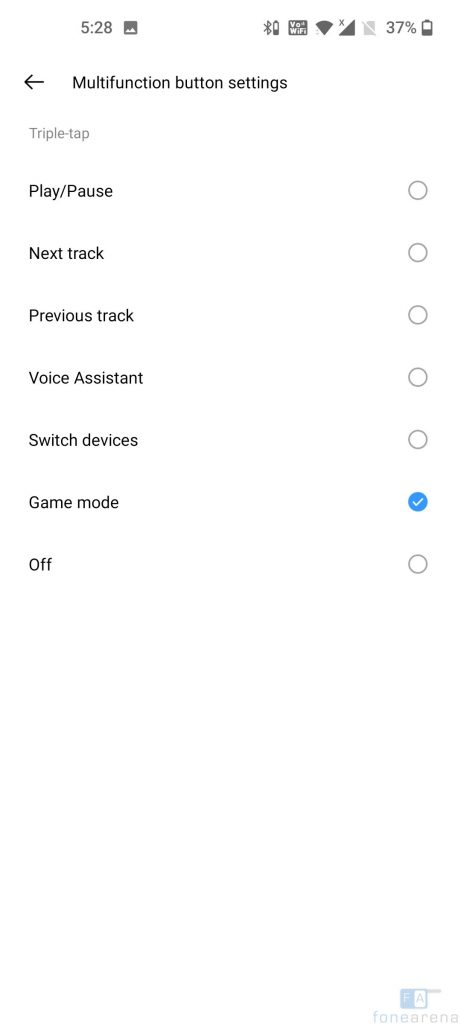Here is a cleaned-up and detailed descriptive caption:

---

This vertical image depicts a smartphone screen with a plain white background, characteristic of a typical device interface. In the upper left corner, the time is displayed as 5:28, accompanied by an icon. The upper right corner is populated with various status icons, including those for Wi-Fi, Bluetooth, battery life at 37%, and signal strength. Below these icons, an arrow points left towards a multi-function button labeled "Settings."

The interface provides instructions in gray for a "Triple Tap," followed by black text commands such as "Play/Pause," "Next Track" (indicated by an open circle), "Previous Track" (open circle), "Voice Assistant" (open circle), and "Switch Devices" (open circle). An option for "Game Mode" is highlighted in blue with a white check mark, while the "Off" option is represented by an open circle. At the bottom, there is a label that reads "For a phone," along with a small identifiable icon above it.

---

This caption provides a clear and thorough description of the image, detailing each element visible on the smartphone screen.